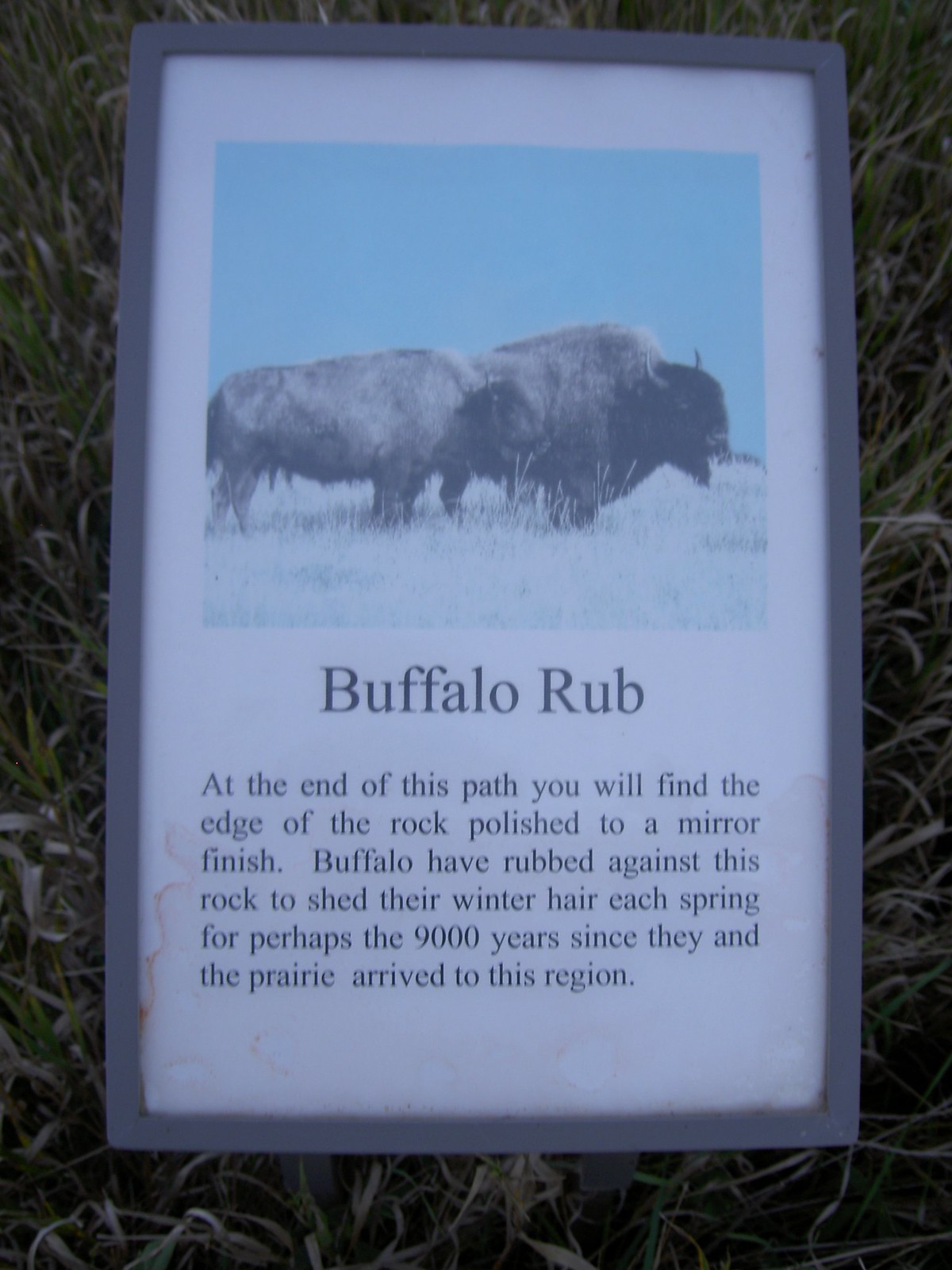This image depicts an outdoor sign or plaque, partially embedded in the ground among grass and dirt. The rectangular sign is enclosed in a gray metal frame, seemingly aged and slightly weathered by exposure, with evidence of sun-fading and soft brown stains at the edges. The upper portion of the sign showcases a vivid color photograph of two large, shaggy buffalo standing side-by-side on a grass plain, set against a blue sky. Both buffaloes have dark heads, manes, beards, and prominent tusks. Below the image, in a white section, there is a title in black text, "Buffalo Rub," followed by a detailed paragraph: "At the end of this path you will find the edge of the rock polished to a mirror finish. Buffalo have rubbed against this rock to shed their winter hair each spring for perhaps the 9,000 years since they and the prairie arrived in this region." This informative sign provides a close-up, descriptive history of the buffalo's interaction with the landscape.